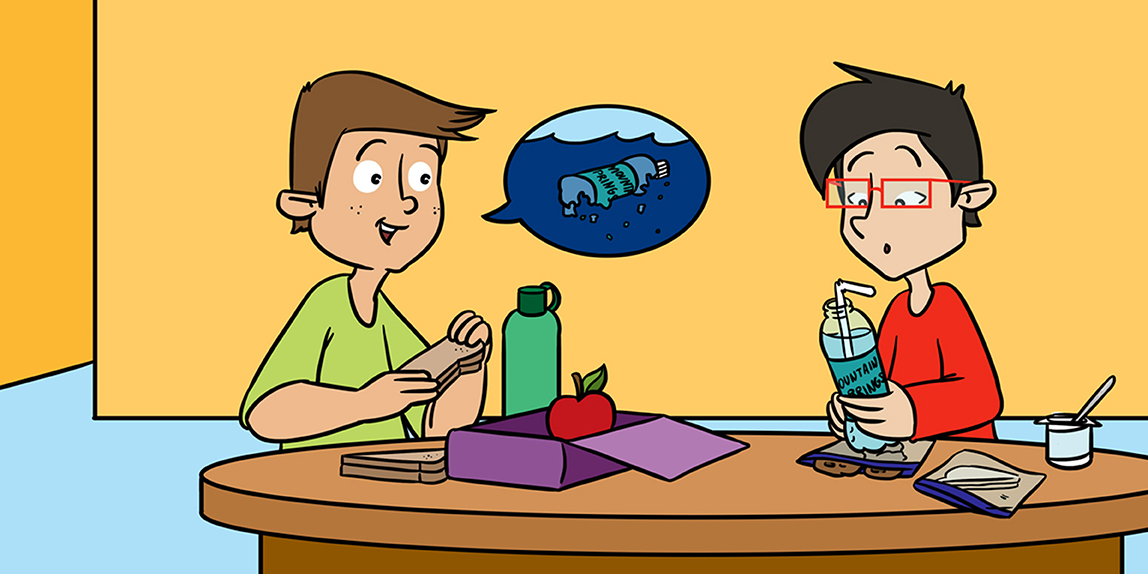The cartoon shows two boys sitting opposite each other at a round table, eating lunch. The setting is a room with pale orange walls and a cyan floor. The scene is drawn in a simple style, with flat colors and no shading. The boy on the left has brown hair, wears a green shirt, and holds a sandwich in each hand. In front of him, he has a purple lunchbox with a red apple inside and a green water bottle. He appears to be talking, as indicated by a speech bubble showing an image of a plastic water bottle floating in the ocean, with waves around it. The boy on the right wears a red shirt, rectangular red glasses, and has darker brown hair. He looks surprised or contemplative as he stares at his own plastic water bottle labeled "Mountain Springs," which has a straw sticking out of it. His lunch items include an half-eaten sandwich in a plastic bag, an empty yogurt container with a spoon, and a bag of cookies. The image evokes a message about the environmental impact of plastic waste.